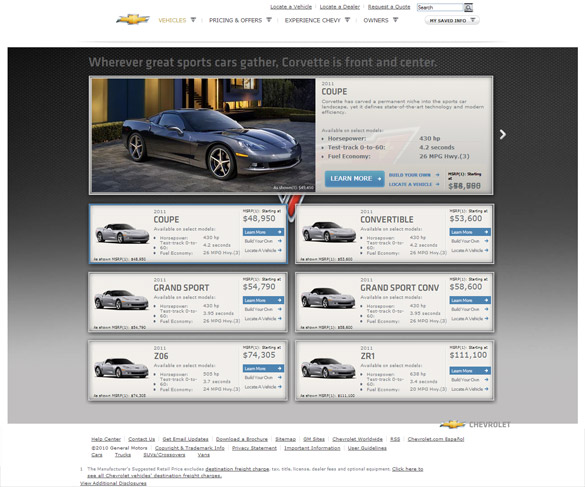In this image, we see a detailed snapshot of a Chevrolet webpage. At the very top, prominently displayed is the Chevrolet logo. Just below the logo, there's a navigation menu featuring buttons labeled "Vehicles," "Pricing & Offers," "Experience Chevy," "Owners," and a "My Saved Info" button. Above these menu options, there are additional categories for "Locate a Vehicle," "Locate a Dealer," "Get a Quote," and a search bar for user convenience.

The main content of the webpage highlights a prominent banner with the slogan "Whenever great cars gather, Corvette is front and center." This is accompanied by an image of a gray 2011 Corvette Coupe, complete with detailed bullet points describing the vehicle.

Further down the page, the layout splits into two columns. Each column contains three distinct car options, each accompanied by their respective images and prices, providing potential buyers with a comprehensive overview of available models.